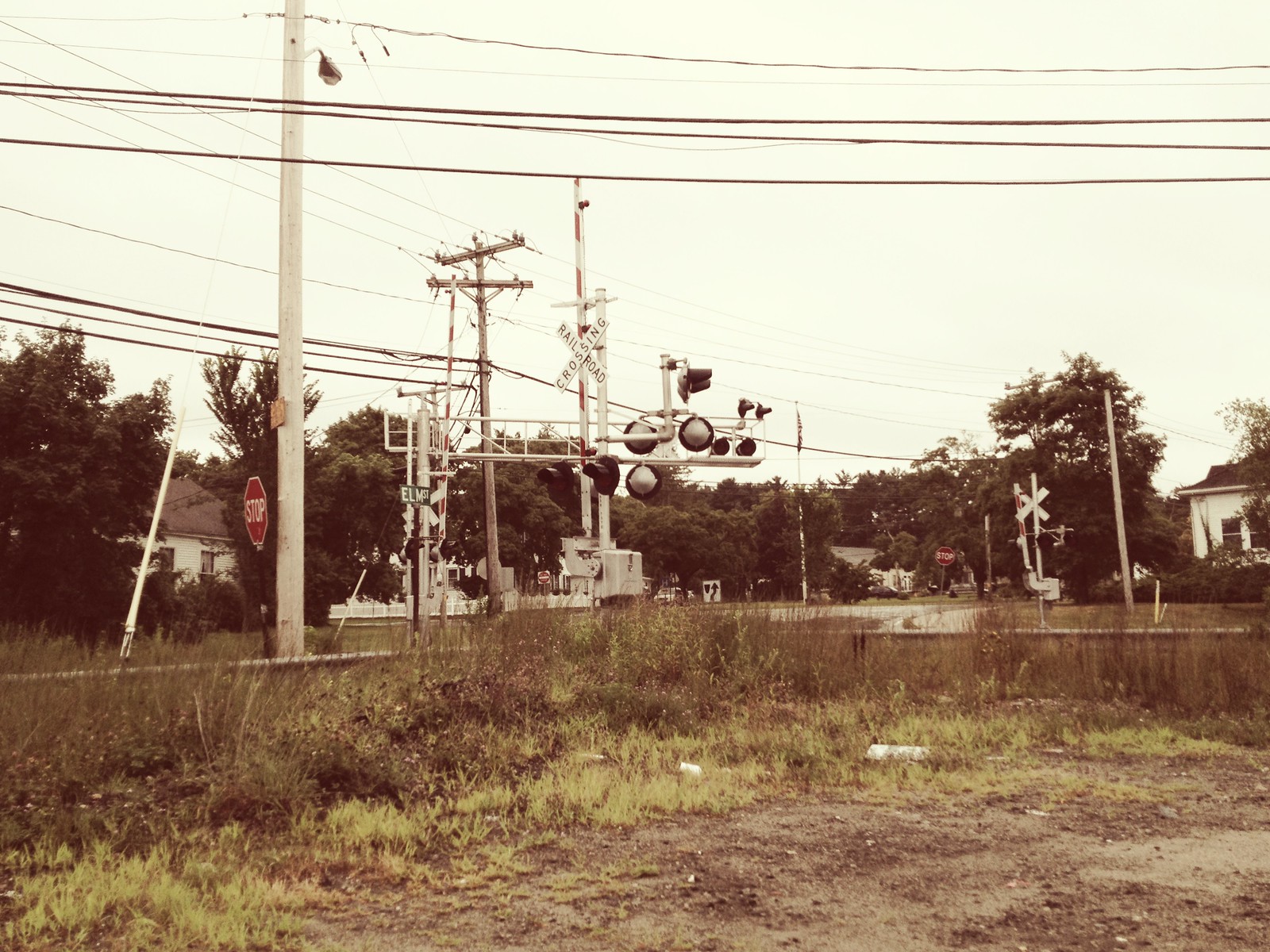The image depicts a vintage-feeling photograph with a yellowish tint, reminiscent of one taken with an older camera. It shows a railroad crossing during the day under a light gray and slightly overexposed sky. The foreground features a field that transitions from mostly bare dirt to taller, brown, and yellowish grass as it nears the road and railroad tracks. The railroad crossing arms, painted red and white, are currently lifted. Overhead, utility lines stretch horizontally, supported by utility poles. In the left-center of the image, a red stop sign is visible. The background reveals a rural neighborhood with white houses that are partially obscured by green-leaved trees and a distant tree line that conceals additional buildings. No people or vehicles are present in the scene, and the overall color palette of the image is muted with dominant grays, browns, and greens.